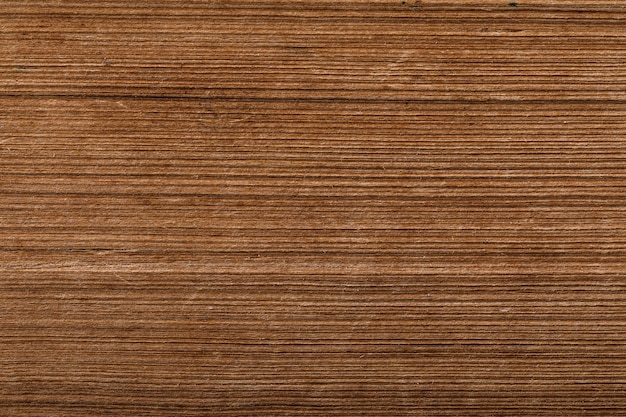The image captures a close-up view of a brown surface, showcasing a variety of wood grain patterns and hues. The surface features an array of lighter and darker brown shades, including elements so dark they are nearly black. The texture includes a prominent darker brown line and several scuffed areas, suggesting wear and tear. The overall look is reminiscent of wood, possibly a table or floor, though some details like thread-like patterns introduce an ambiguity that could also be interpreted as fabric, possibly corduroy. However, the predominantly wood-like characteristics, inclusive of the grain and scuffing, lean more towards a wooden surface that might be intended for refinishing, highlighting areas needing repair.